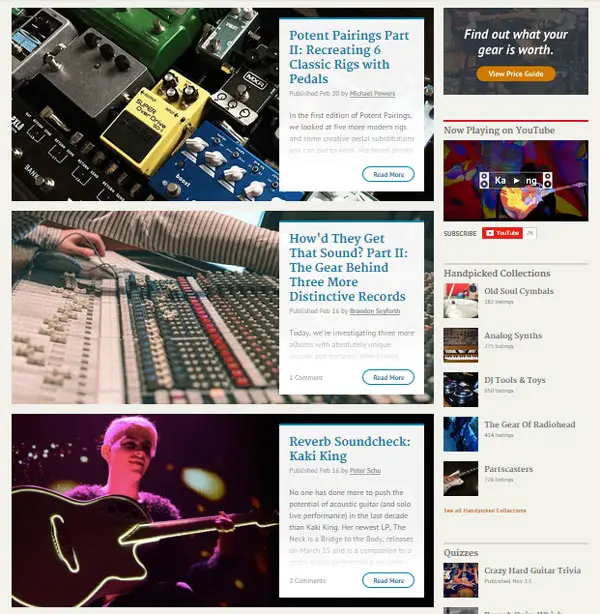Sure, here is a cleaned-up and detailed caption for the image:

---

The screenshot depicts an online music magazine page with several featured articles. The top article, titled "Potent Pairings Part 2: Recreating 6 Classic Rigs with Pedals," is prominently displayed with the headline in a bold blue font. Accompanying this article are vibrant pictures of gear in various colors—blue, yellow, green, silver, and black—each adorned with small pig icons, though their exact purpose isn't clear.

Below, the second article titled "How'd They Get That Sound Part 2: The Gear Behind 3 More Distinctive Records" also has its headline in striking blue. Next to this, there is an image of a man's arm interacting with sound control equipment, adding a tactile dimension to the content. Both articles feature "Read More" links in blue for further reading.

The third article, located further down, is titled "Reverb Soundcheck: Cocky King," again in blue text, with an adjacent "Read More" option. Beside this is an image of a man holding a guitar, wearing what appears to be a dark-colored, likely purple, shirt. The background is dark, highlighting the illuminated guitar and the glowing lights behind him, creating a dramatic effect.

The right-hand side of the page is populated with advertisements, quizzes, and recommendations, providing additional interactive content for the reader.

---